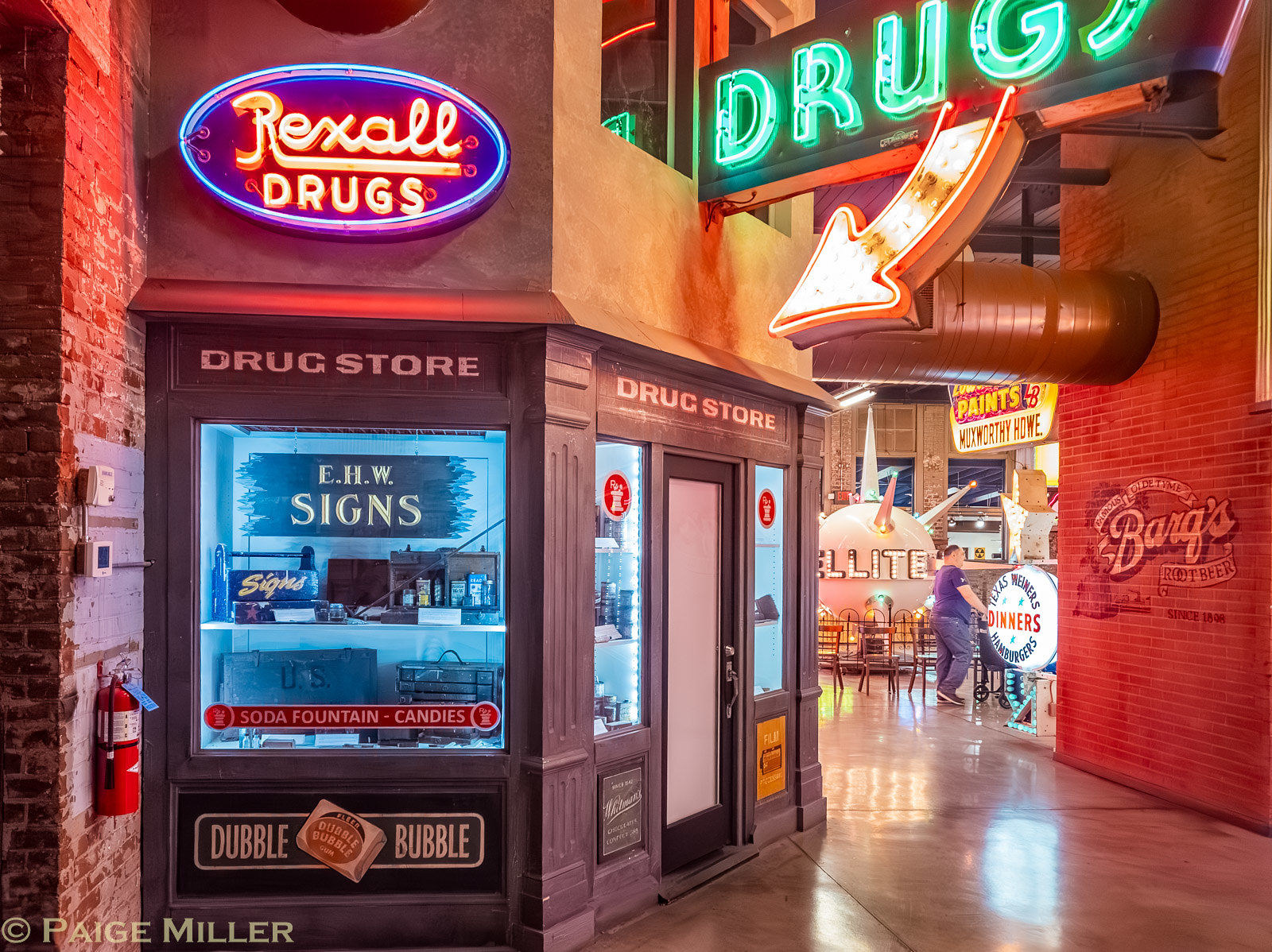This photo captures the interior of a large, well-lit venue that appears to display vintage themes, possibly part of a museum exhibit focused on neon signs. On the left side, there is a mock-up of an early 1900s drugstore storefront with a neon sign that reads "Rexall Drugs" in a purple oval. Below it, the storefront window showcases phrases like "Soda Fountain" and "Candies," along with a small Double Bubble gum advertisement in the bottom left corner. This window is said to have a transparent blue tint with some visible bags inside.

Prominently displayed above the entrance to the drugstore is a larger green neon sign reading "DRUGS" with a red arrow pointing down to the doorway. Adjacent to the drugstore, on the far right wall, there is an image of a Barks Root Beer logo down a hallway, suggesting more vintage displays beyond. Additional details include a white neon circle sign that reads "DINNERS" and a fire hydrant mounted on the left side of the building. The scene is completed with some tables and chairs where a person in a purple shirt and jeans can be spotted, adding a touch of life to the nostalgic setting.